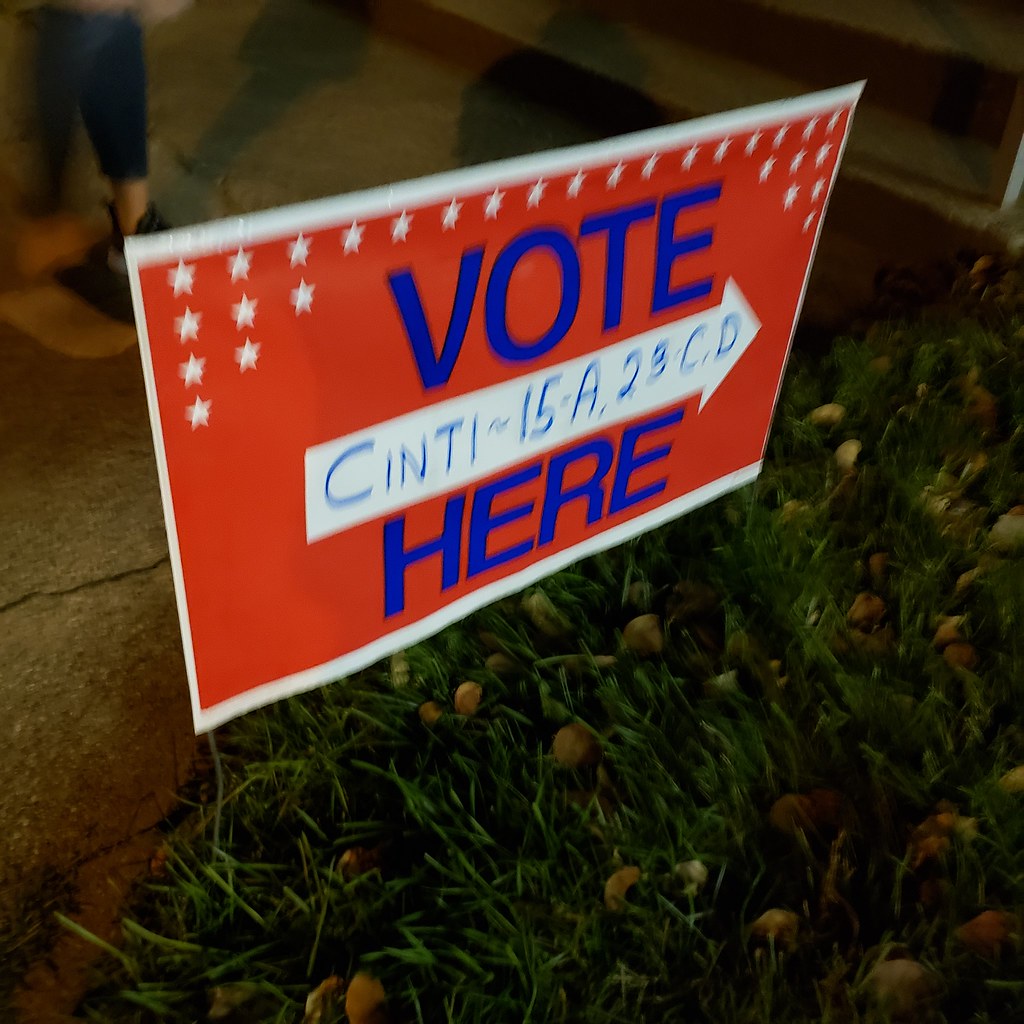This image captures a nighttime scene with a blurry photograph of a colorful sign partially obscured by grass and scattered leaves. The sign, held in place by two metal prongs, is prominently red with a white border and adorned with numerous white stars along the top edge. The main text on the sign reads "Vote Here" in large blue letters. Separating the words "Vote" and "Here" is a white arrow pointing to the right, inscribed with "Cinti-15A 23C D" in blue text. On the left side of the image, there is a small stone walkway where the legs of a person, possibly a woman dressed in tight jeans and black sneakers, are visible. The indistinct upper left corner of the photo suggests a darker sky, adding to the overall impression that the scene is set outdoors at night.